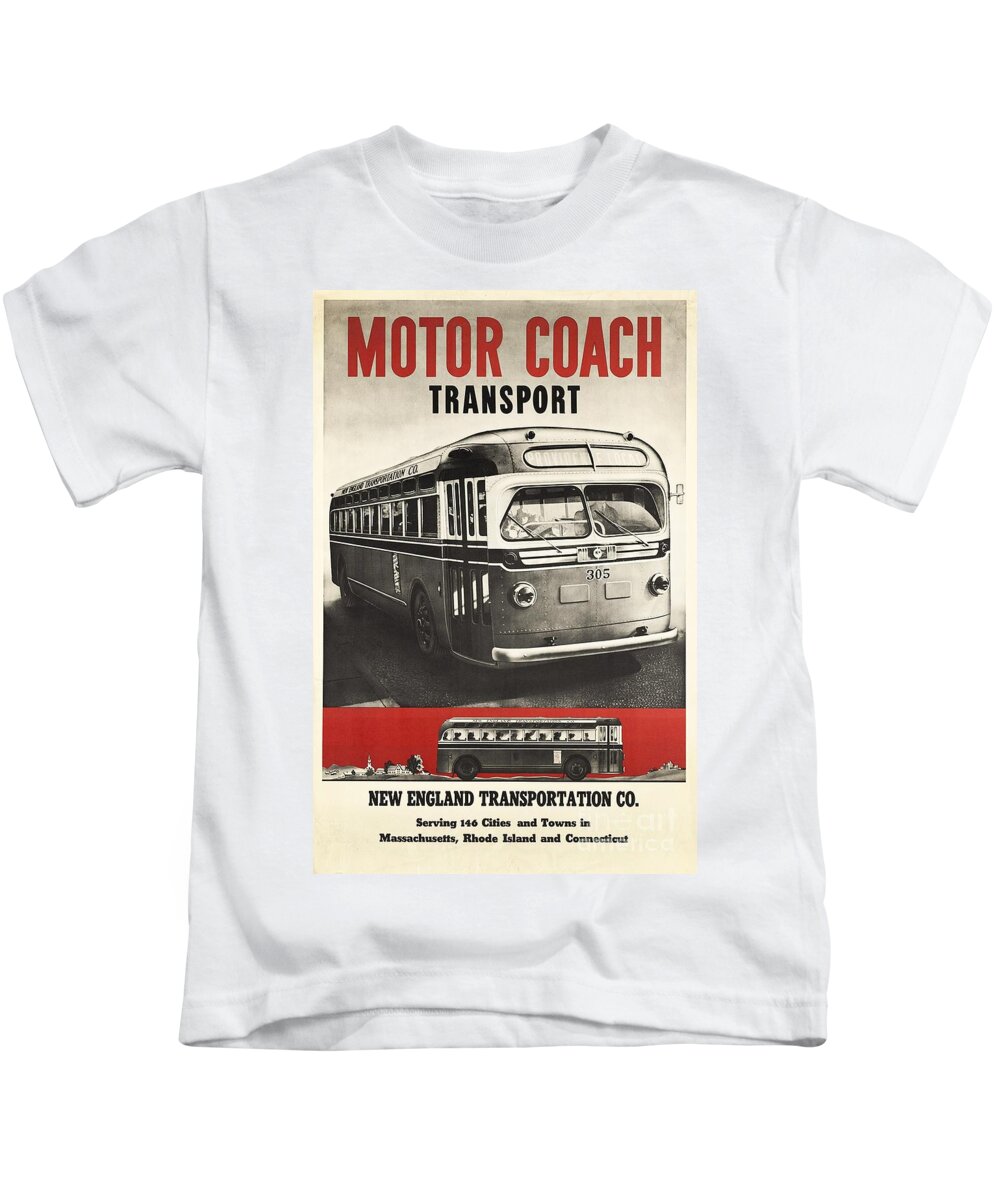The image showcases a white crew neck t-shirt set against a pure white background, resembling a clipart or advertisement photo. The main feature of the t-shirt is a large rectangular graphic printed on the front, comprising a vintage, black-and-white theme with the headline "Motor Coach" in red letters at the top and "Transport" in black letters directly below. The central part of the graphic displays a vintage motor coach bus facing forward, identified by the front windows, a slightly whited-out text, and headlights. The number "305" is visible on the center of the bus. To the left of the front, there is the bus's entrance door, which is mostly white at the top and black at the bottom, along with the front wheel extending to the back corner. Beneath this central image, there is another depiction of the motor coach viewed from the side, with people visible inside, set against a cream-colored background. The lowest part of the graphic features text in black that reads, "New England Transportation Company serving 146 cities and towns in Massachusetts, Rhode Island, and Connecticut." The overall design employs muted cream, red, and black-and-white tones, emulating the feel of a retro poster artfully printed on the t-shirt.